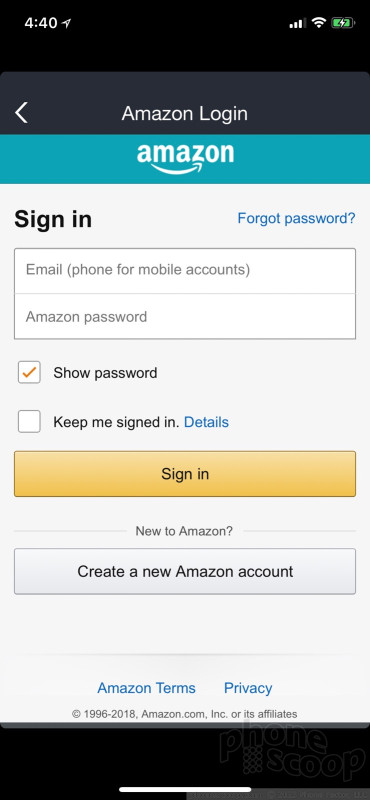This image is a mobile screenshot displaying the login page for Amazon. It may be from the Amazon app or accessed through a mobile browser, identifiable by the tall rectangular shape and the presence of icons at the top of the screen, including indicators for battery life, Wi-Fi signal, cellular data signal, and the device's current time.

At the top, a navy blue bar features the white text "Amazon Login" and includes a back arrow on the left side, allowing users to return to the previous page. Directly below, a light blue banner showcases the Amazon name and logo in white. The background of the sign-in section is a light gray color.

Within the sign-in area, "Sign in" is prominently displayed in black text, accompanied by a "Forgot password" link in blue text for users who need to reset their passwords. Underneath this section, there are two input fields: the first for entering an email address and the second for inputting the password. Below these fields are two checkboxes: one labeled "Show password" and the other "Keep me signed in." Completing the sign-in section is a yellow "Sign in" button.

Finally, at the bottom of the login form, there is a gray button for users who need to create a new Amazon account.